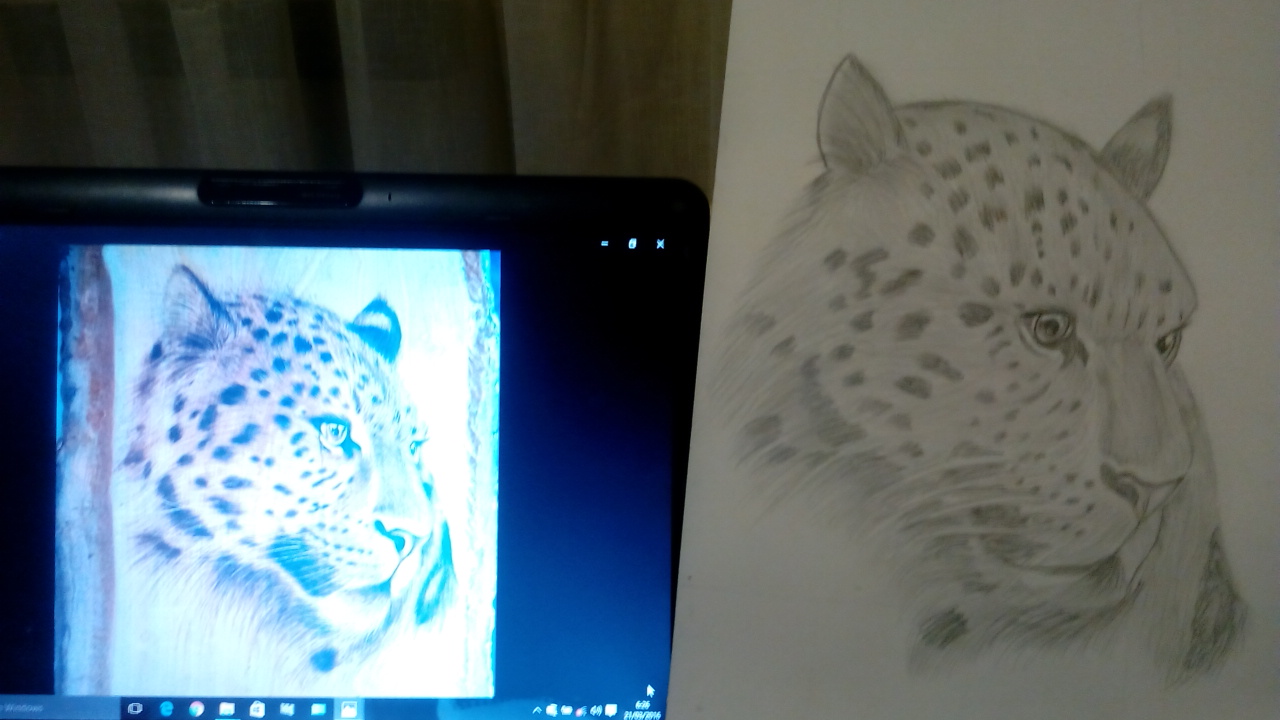A detailed comparison of two images, both depicting a beautifully spotted jaguar, set against a gray backdrop. On the right, a meticulously sketched, monochromatic drawing of a jaguar captures the animal's stunning details, with distinctive spots, expressive eyes, small ears, and a long nose. The sketch is done on a piece of white paper standing upright, showcasing the artist's skill in rendering realistic features. On the left, a black tablet displays a digital image of the same jaguar's head, highlighting its natural beauty with vibrant detail. The tablet's screen background is blue, and beside the jaguar's image, there's a hint of a tree limb, enhancing the lifelike quality. The juxtaposition of the hand-drawn sketch against the digital rendering provides a fascinating comparison, emphasizing the jaguar's elegance and the artist's talent in both mediums.